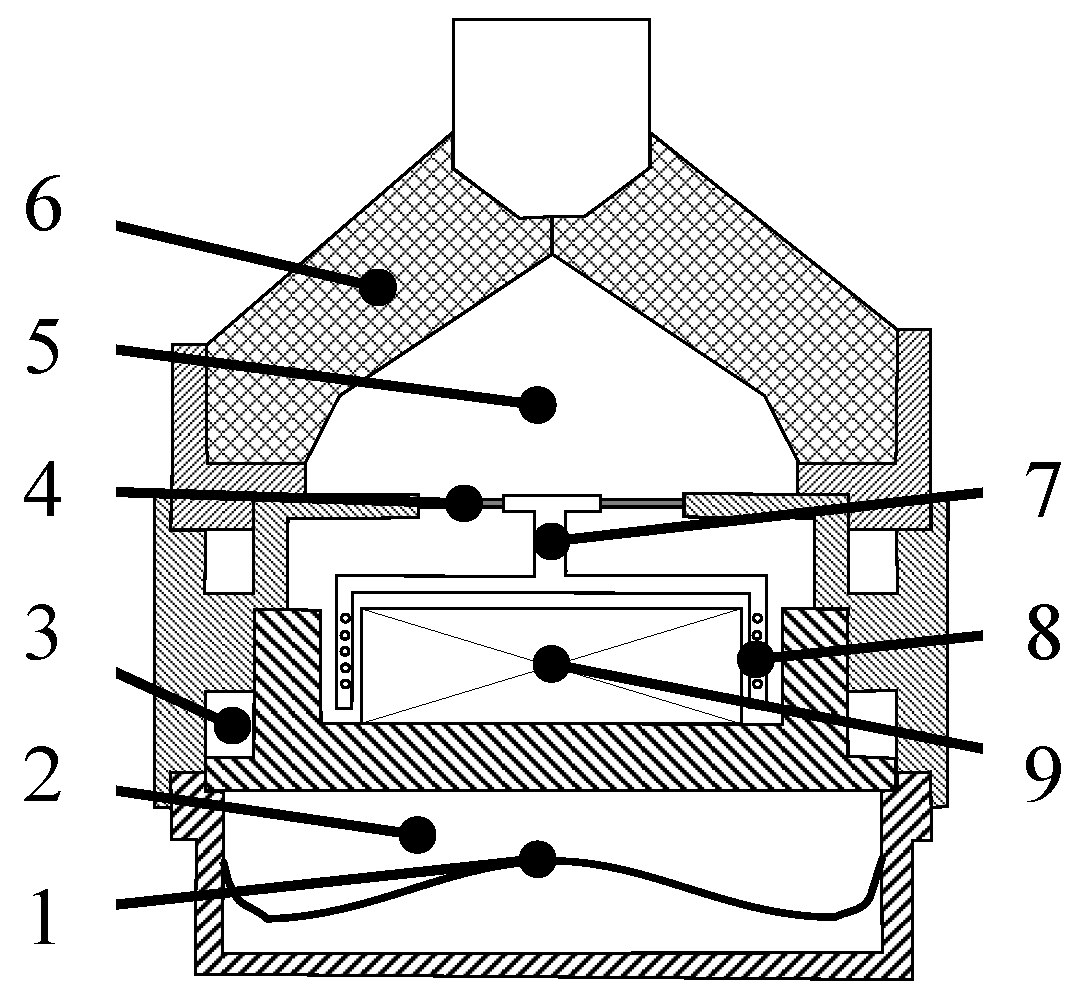This image is an intricate black-and-white diagram, resembling an unlabeled schematic or cross-section, featuring the numbers 1 through 9 pointing to various parts of the illustration. The numbers are distributed uniquely: along the left side, numbers 1 through 6 are arranged in reverse order from bottom to top, while on the right side, numbers 7 through 9 are ordered sequentially from top to bottom. Each number is connected by a line ending in a dot, intended to indicate specific components or areas within the diagram, which are currently unspecified. The diagram itself is adorned with a variety of black-and-white patterns and textures that differentiate its sections—examples include small and large diagonal lines, both right-leaning and left-leaning, cross-hatching, and graph paper-like squares at the top. The entire illustration maintains a square-like overall shape, potentially suggesting a boxy structure, and the exact purpose or subject of the diagram remains unknown due to the absence of labels or a key.